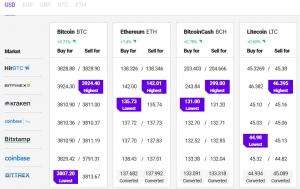The image depicts a website or app interface designed for tracking stock indexes and cryptocurrency indexes, presented in a small, landscape-oriented photo. The interface is set against a gray background with a white top border. 

In the top portion of the interface, there is a white section containing various options. On the left, a column lists different currencies, starting with "USD" (U.S. Dollars) highlighted in pink. Other currency options include "EUR" (Euros), "GBP" (British Pounds), "BTC" (Bitcoin), and "ETH" (Ethereum). 

Below this, a gray box is segmented by white columns that organize different stocks or cryptocurrencies. The first column features "Bitcoin" at the top, with various numerical data below it related to buying and selling, including a "buy" column and a "sell" column. Notably, two of these numbers are highlighted in purple, one in each column. 

Next, "ETH" (Ethereum) is listed with a similar format for buying and selling data, also with one number highlighted in each column. Following Ethereum are "Bitcoin Cash" and "Litecoin," each structured similarly with their respective data columns.

To the left of these columns, against the gray border running horizontally, there are listings for different exchanges where these cryptocurrencies can be traded.